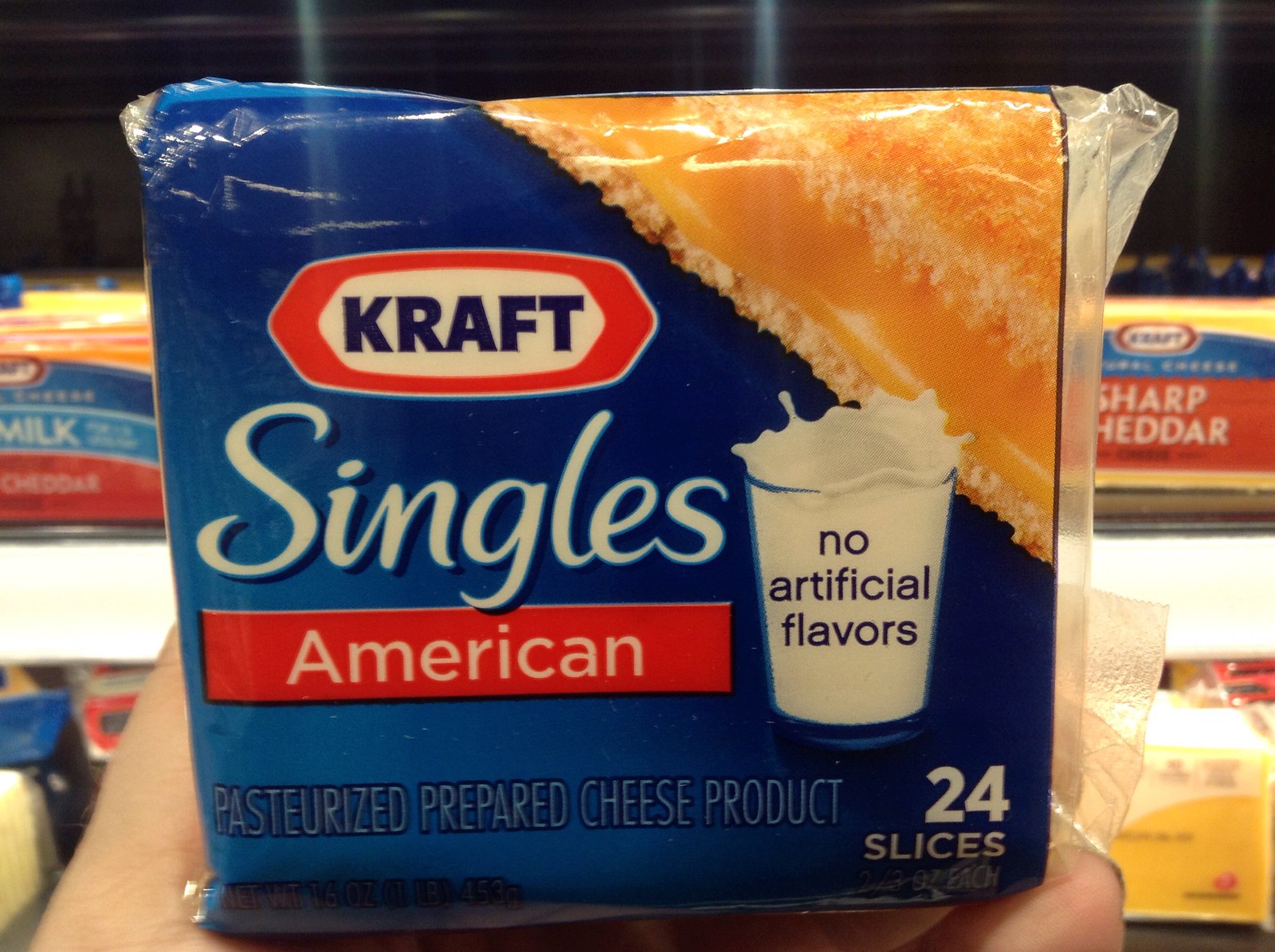This landscape photograph captures a moment in the cheese refrigerated section of a grocery store. At the forefront, a person holds a package of Kraft American sliced cheese. The package prominently displays the Kraft logo at the top, followed by the word "singles" in a cursive script. Below this, the flavor "American" is clearly indicated. To the right of the flavor description, a stylized glass of milk is featured with text proclaiming "no artificial flavors." Lower down, in light blue text, the package specifies that it contains "pasteurized prepared cheese product." In the bottom right corner, the package notes that it includes "24 slices." The vibrant array of various other cheeses on adjacent shelves creates a busy and colorful backdrop, reinforcing the grocery store setting.